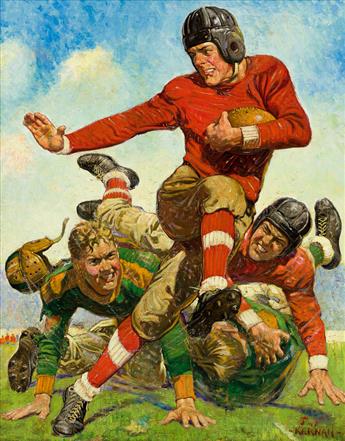The image is a detailed, vintage painting by Joseph F. Kernan titled "Object of Desire," which served as the cover for the 1932 edition of the Saturday Evening Post. The artwork captures an exciting moment in a college football game, characterized by its old-fashioned aesthetic. At the center of the scene, a football player in a red long-sleeved sweater, brown khaki football pants, and red and white striped socks is sprinting with the football tightly clutched in his arm. His black leather helmet sits firmly on his head, contrasting with the modern hard helmets.

The painting vividly portrays the action on the field: the player is mid-stride with one foot on the ground and the other knee raised high. Behind him, several opposing players in green uniforms are diving in a desperate attempt to tackle him. Their leather helmets have flown off, one player's face contorted in a grimace as he lunges forward. Another teammate of the ball carrier is seen taking down two of these opposing players.

The background features a vibrant green football field extending towards a blue sky dotted with white, fluffy clouds, adding to the nostalgic feel of the scene. The colors used in the painting are predominantly red, tan, green, blue, and white, which enhances the dynamic and lively atmosphere of the moment captured in this timeless piece of sports art.